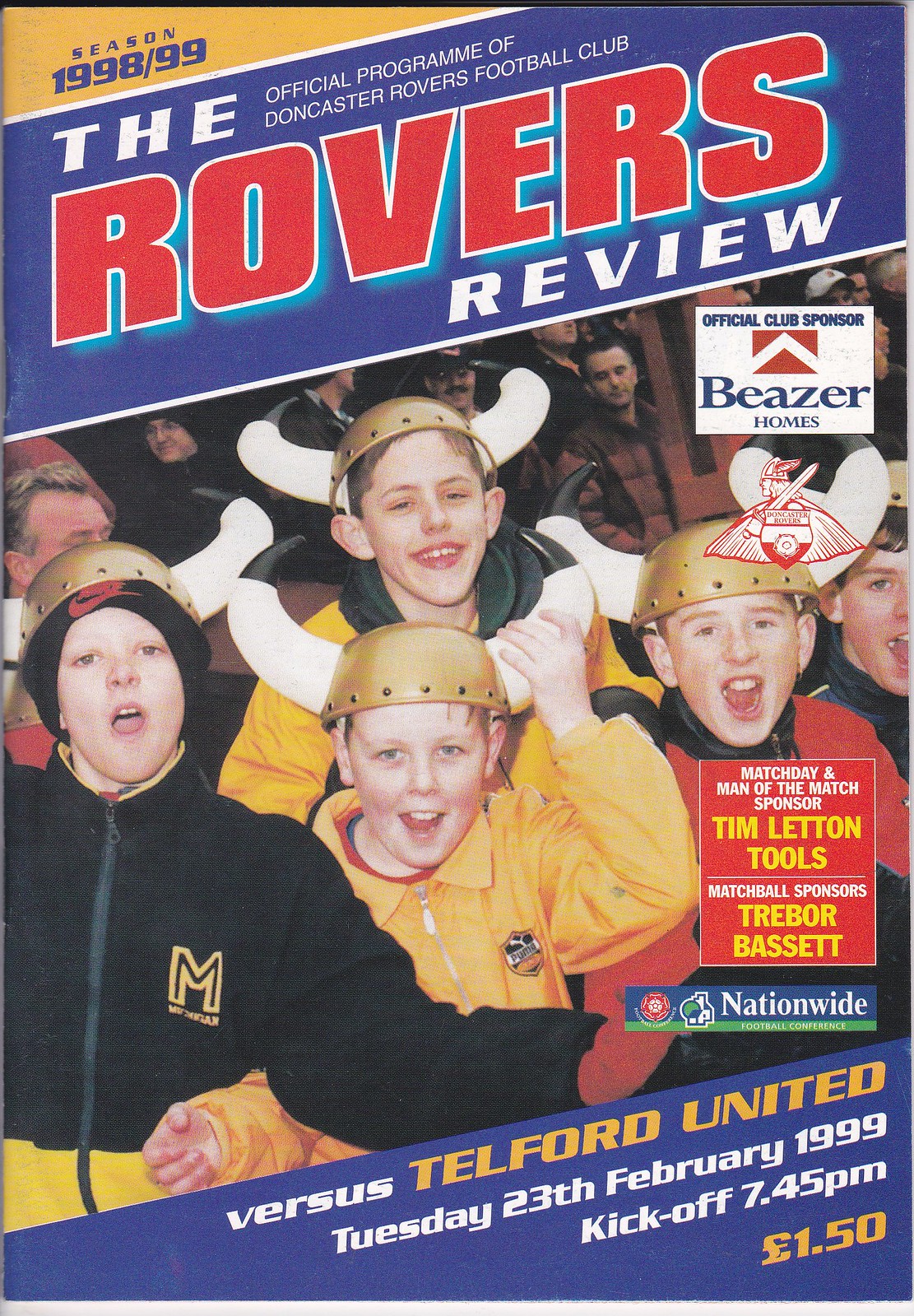The image showcases a detailed cover of the Official Program of the Doncaster Rovers Football Club for the season 1998-99. Dominating the top left corner is a gold triangle with a white bottom outline that distinctly marks "Season 1998-99." Adjacent to this, a prominent blue banner displays "The Rovers" with "The" in white and "Rovers" in bold red text, followed by "Review" in white, indicating this is the titular Rovers Review. Above the banner, in a smaller, yet noticeable font, it reads, "Official Program of Doncaster Rovers Football Club."

The central portion of the cover features a vibrant group of children, estimated to be between 8 and 12 years old, wearing celebratory Viking helmets in gold with large, soft white horns. They appear jubilant and engaged, embodying the enthusiasm of the event.

Below the children's image, another blue banner stretches across the page, stating the specifics of the match: "Versus Telford United, Tuesday, 23rd February 1999, kickoff, 7.45pm," followed by the program price of £1.50. 

On the right center section, the logo of the official sponsor, Beezer Homes, is prominently displayed. Below this logo, a stylized red depiction of a Viking holding a sword over a shield encapsulates the team’s emblem. A red box beneath this emblem highlights the "Match Day and Man of the Match Sponsor," Tim Letton Tools, and further down, "Match Ball Sponsors," Trevor Bassett. Finally, at the bottom, the Nationwide Football Conference logo is positioned, reaffirming the official nature of the program.